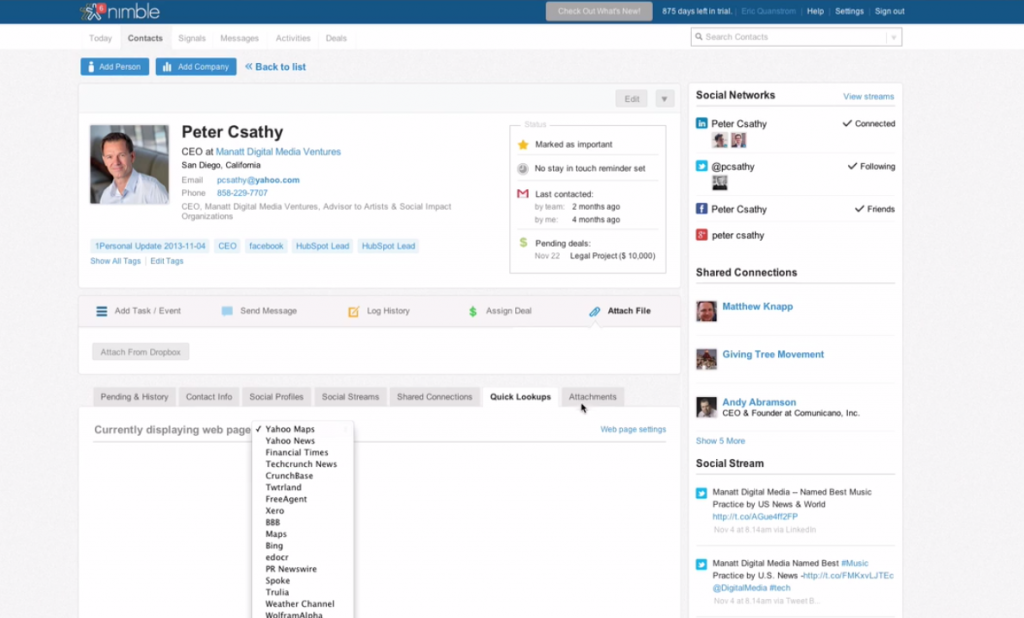The image depicts a website designed for business networking, reminiscent of LinkedIn, named Nimble. In the top left corner, the site's name "Nimble" is displayed alongside its emblem, which resembles a five-point open star. The website's navigation bar at the top includes several tabs: "Today," "Contacts," "Signals," "Messages," "Activities," and "Deals," suggesting it offers various functionalities potentially including sales-related features. Additional options, such as a help section and sign-out button, are also present along the top.

Dominating the main section of the page is a profile featuring a picture of a gentleman named Peter Csathy, whose name is spelled out as C-S-A-T-H-Y. He is identified as the CEO of Digital Media Ventures, based in San Diego, California. His biography, complete with contact details including email and phone number, and his titles such as CEO, advisor, and social impact organizer, are prominently displayed to the left of his photo.

Below his bio, a series of updates and clickable links provide further information about his activities and engagements. Tags indicate his presence on various platforms, such as Facebook. To the right of his profile, a section highlights his connected social networks, offering further insight into Peter's digital presence and professional affiliations.